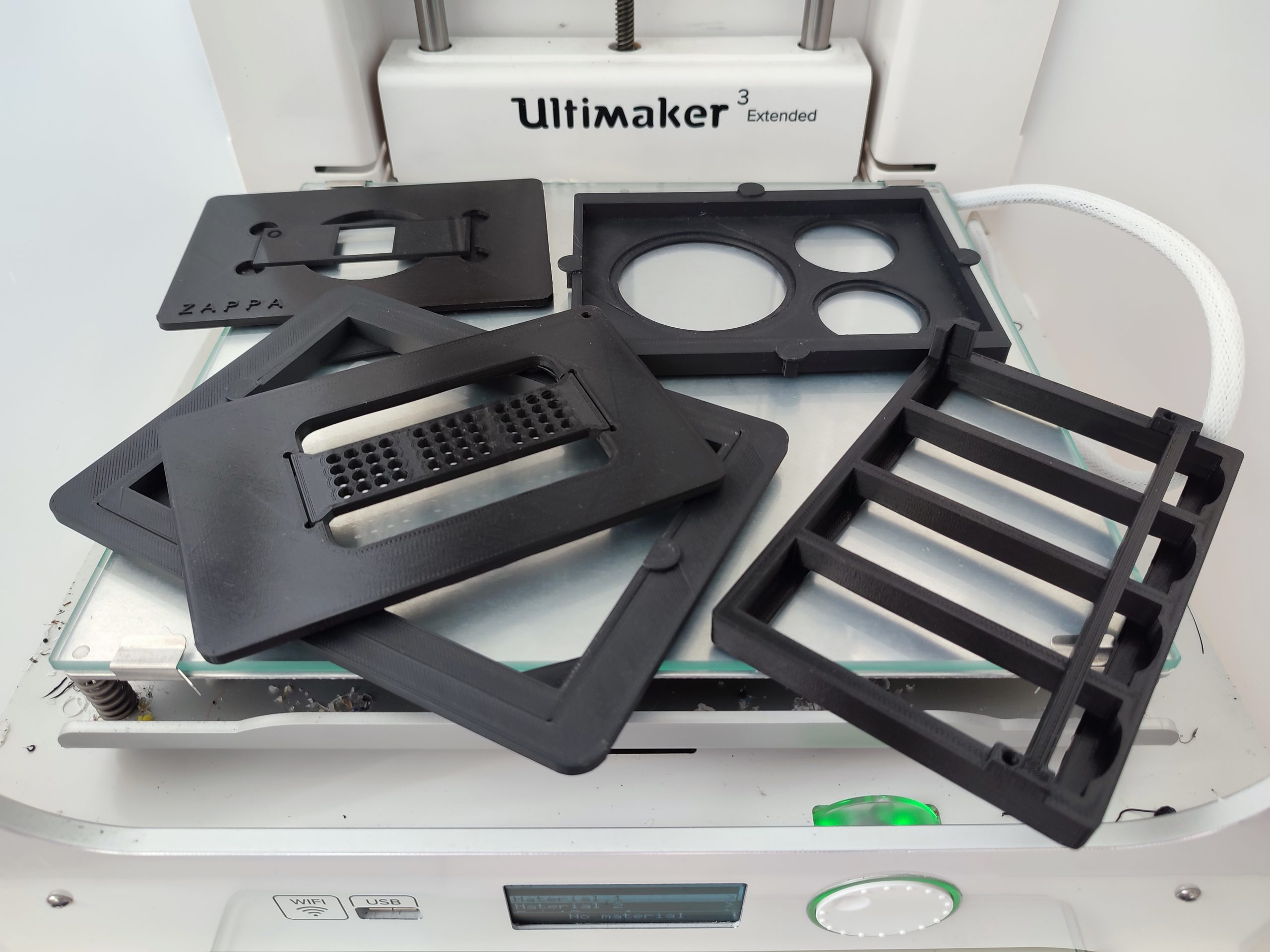The image depicts a disassembled Ultimaker 3 Extended 3D printer that is primarily white with a tan hue. The top of the device prominently displays "Ultimaker 3 Extended" in black text. The front of the printer features a white dial with a green surrounding layer, partially visible through a reflective glass surface commonly seen in traditional printers. Placed on the glass surface of the printer are multiple black, plasticky structures of varied designs and shapes. Among these pieces, one tray has three circular cutouts, another has three middle slots and hollowed sections, and another features a pattern resembling a keypad with small dots. These varied black components appear essential for the functionality of the printer, though the exact configuration of the machine is not entirely clear from this angle.